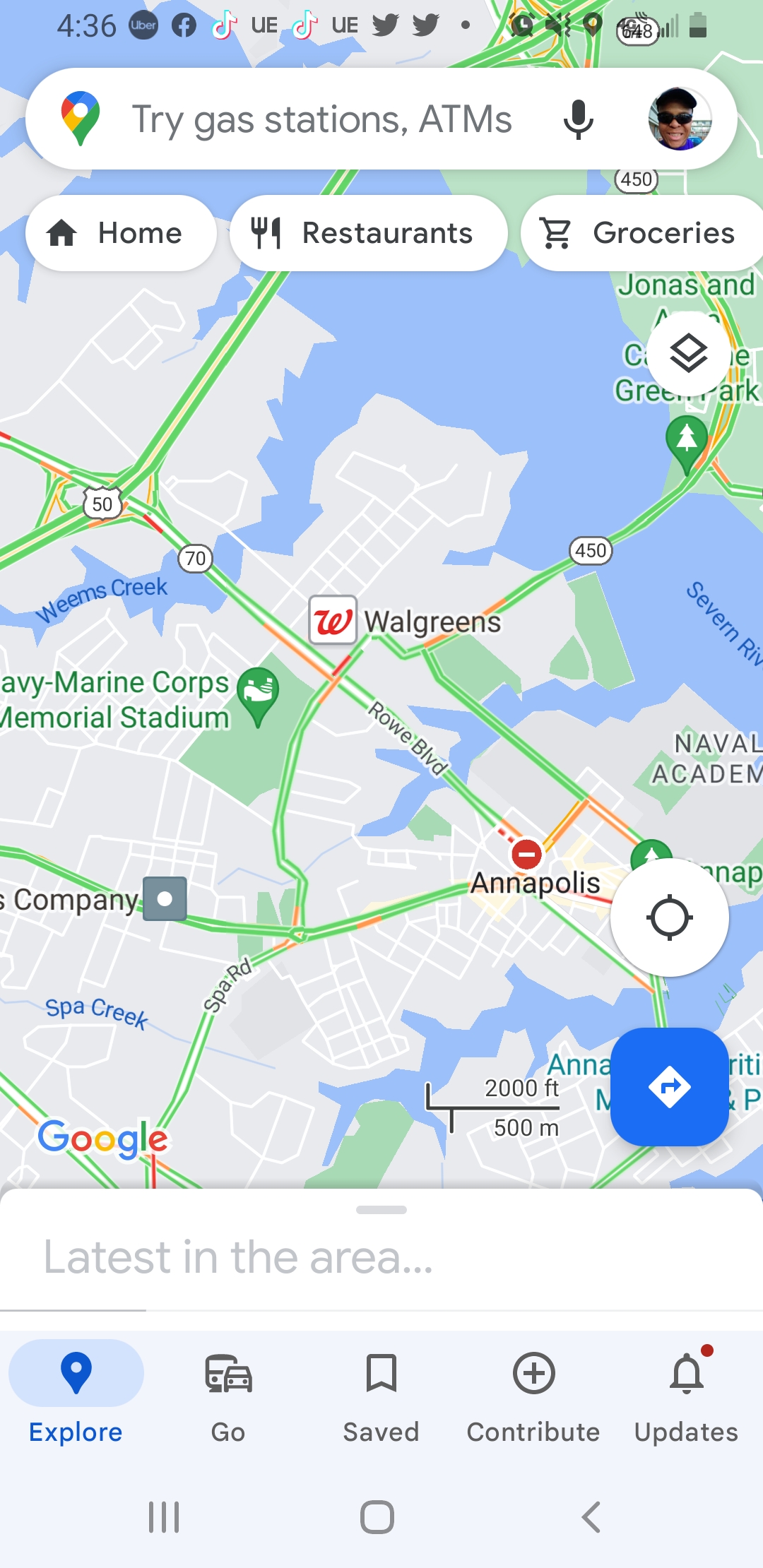This is a screenshot taken from a mobile phone displaying Google Maps. At the top, the device shows various notification icons, including alerts for Twitter, TikTok messages, and Facebook, with the time indicating 4:36 and the battery at one-third full. Below this, the search bar prompts to "try gas stations, ATMs" and displays a microphone icon alongside a smiling black man in a black beret and black sunglasses, representing the user's Google account. The map highlights Annapolis, featuring landmarks such as a Walgreens, the Naval Academy, Navy Marine Corps Memorial Stadium, and various roads and waterways. At the bottom, the toolbar offers options to "explore," "go," "saved," "contribute," and "updates."